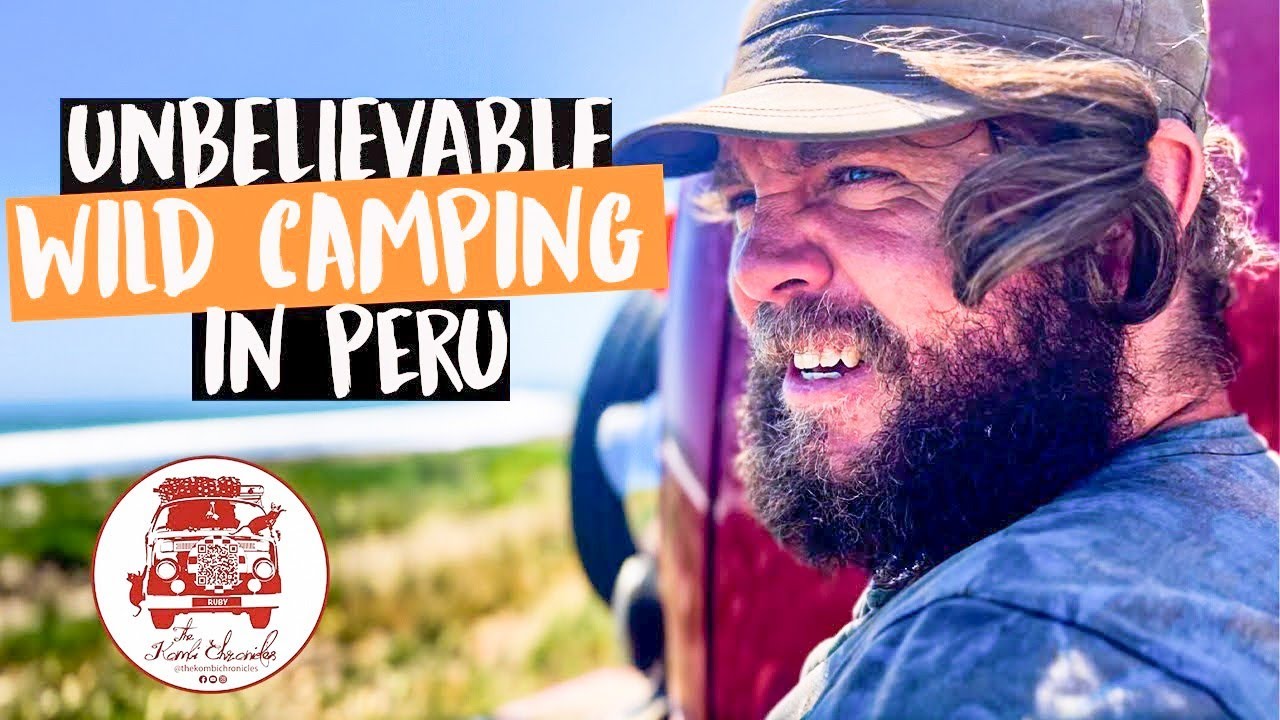The image appears to be a thumbnail for a YouTube video or an advertisement, prominently featuring the caption "UNBELIEVABLE WILD CAMPING IN PERU." The text is in a marker-style font, with "UNBELIEVABLE" and "IN PERU" in white against a black background, while "WILD CAMPING" appears in white against an orange background. On the left side of the image, there is a logo and social media icons at the bottom. The right side displays a man with a thick beard and wavy hair, wearing a green hat and a blue shirt. His hair is being blown back by the wind, hinting at a dynamic or distressing situation as he gazes intently into the distance, possibly squinting against the sun. Behind him, there's some form of vehicle with a spare tire, and the background includes a grassy area and a distant shoreline, adding to the adventurous vibe of the scene.